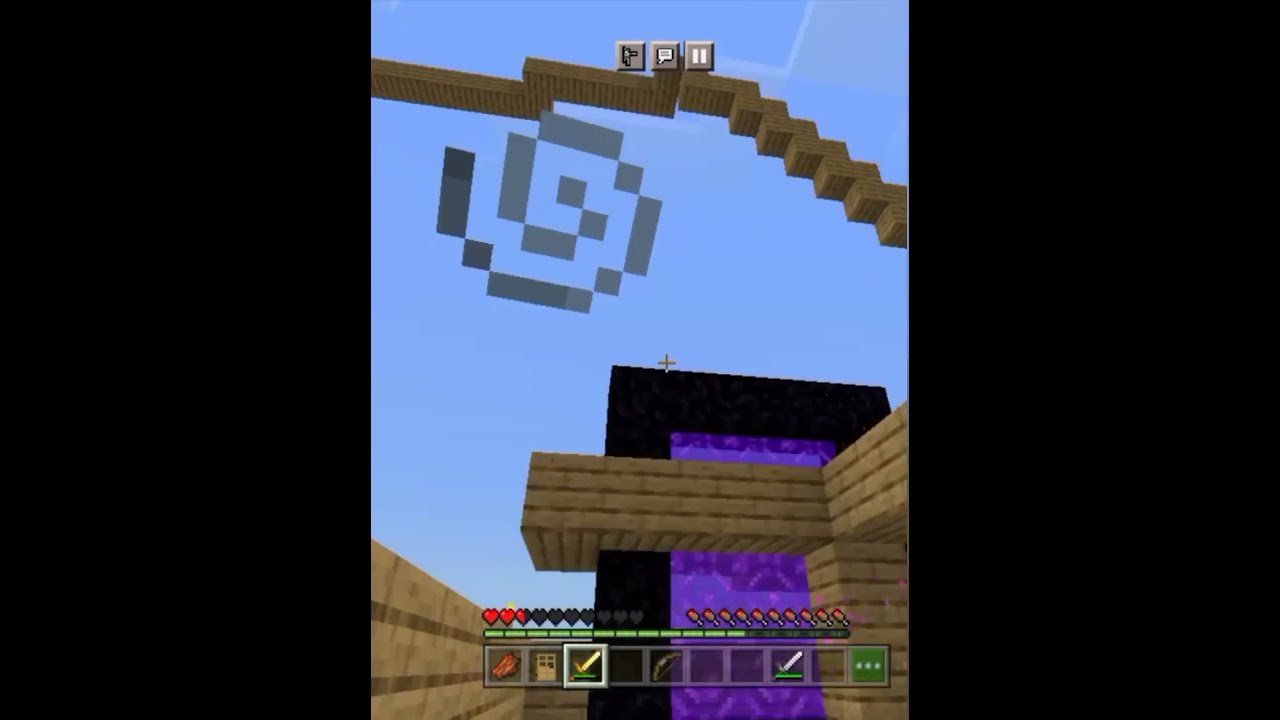The screenshot from a video game features a vertically oriented, rectangular gameplay area flanked by wide black stripes on both sides. The image is highly animated and carries a cartoonish aesthetic reminiscent of games like RuneScape or Minecraft. In the center, there is an intricate setup involving brown brick architecture. This brick structure begins from the bottom and spirals upwards in a staircase-like fashion, wrapping around a central, black-bordered purple portal.

Amidst a bright blue sky, three gray cubes hover at the top. Each appears to have distinctive symbols: a drill, a chat box, and a stop sign, respectively. Below this section, there's a gray swirl and a bridge aligning with the brick stairs.

At the bottom of the image, a user interface displays multiple interconnected boxes. These include icons representing various items: bacon, a door, a checkmark, a bow and arrow, a sword, and a green box with ellipses. Additional UI elements consist of a green health bar paired with red hearts, and what might be roses on the right-hand side.

Overall, the design showcases an engaging blend of architectural and interface elements placed against the vibrant backdrop of a beautifully animated sky.